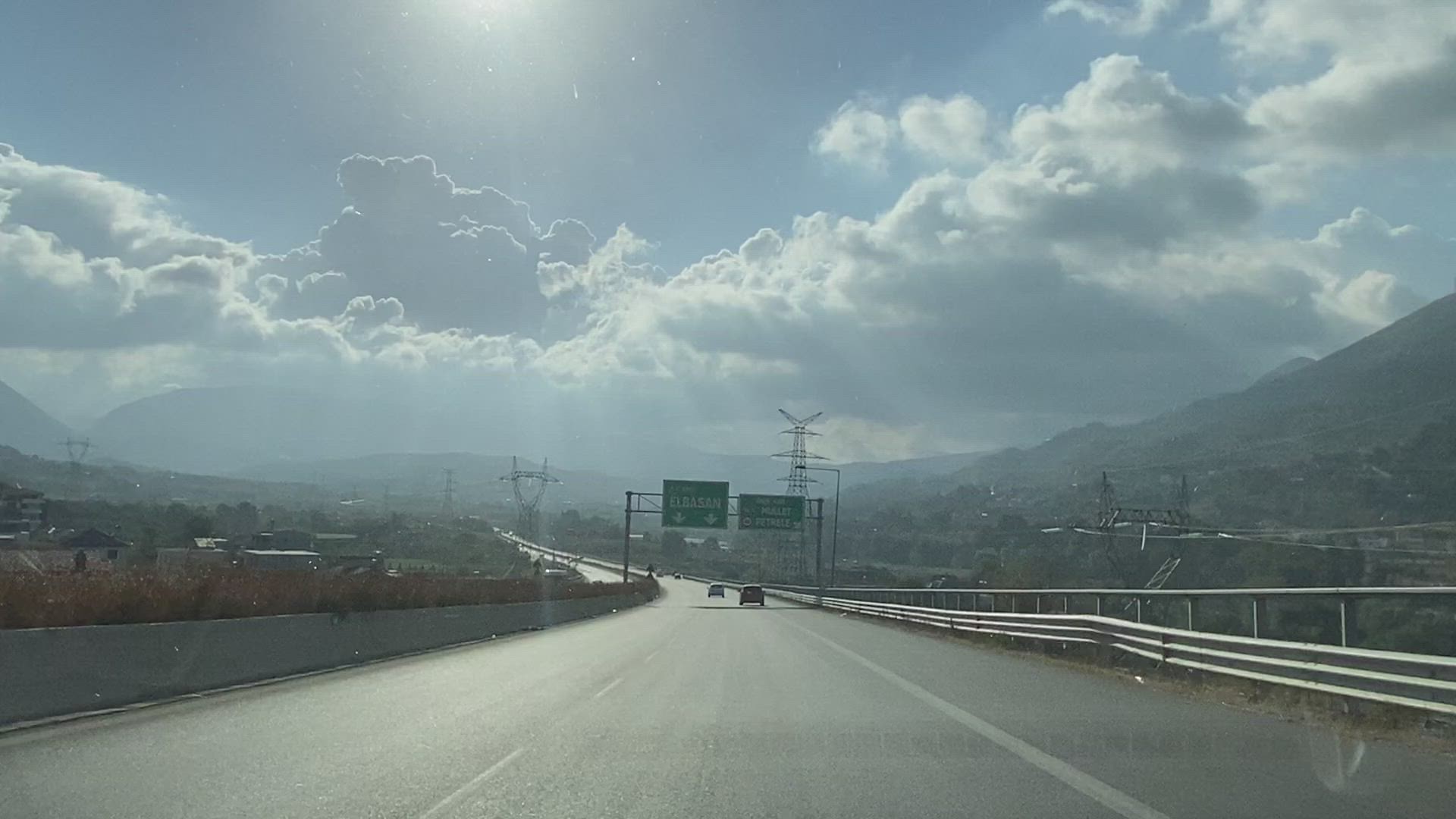A photograph taken from the center of a highway reveals a broad, open road stretching into the distance. The perspective suggests the image was captured from a moving vehicle. Far off in the distance, two large green and white highway signs are mounted on a robust metal structure, anchored by poles on either side of the road. The details on the signs are unreadable due to the image's quality and distance. Flanking the highway, a sturdy guardrail runs parallel to the asphalt, beyond which lies a fence. The roadside is lined with a dense array of bushes. To the right of the image, a distant mountain range is partially visible, while to the left, more mountains recede into the background. Dominating the sky, tall silver electrical towers punctuate the horizon, and a clear blue sky with the sun softly peeking through adds a serene backdrop to the scene.